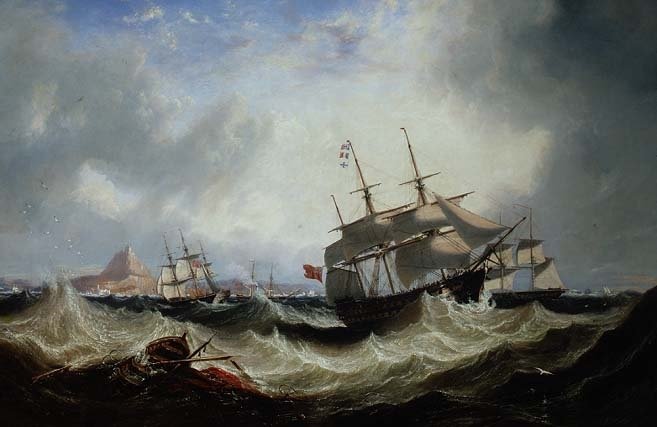This detailed oil painting, titled "Shipping Off Gibraltar in Heavy Seas" by John Wilson Carmichael, is a dramatic seascape capturing a fleet of ships struggling against fierce, towering waves near the shoreline. The scene is dominated by a large three-masted sailing vessel at the center-right, its white sails bravely raised amid a dark, turbulent ocean. Surrounding this main ship are several other clippers with black and white sails, battling the same treacherous waters.

In the bottom left corner, a small lifeboat appears precariously close to being overwhelmed by the crashing waves. Seagulls circle the scene, adding to the chaotic atmosphere. The ocean's palette of blue, gray, and white underscores the severity of the brewing storm, which is further emphasized by the black storm clouds encroaching from the right side of the canvas.

The sky occupies the top two-thirds of the painting and features a tumultuous blend of dark, menacing clouds and a slight bluish tint, hinting at the ongoing struggle between the storm and the receding daylight. In the background, a stone mountain and structures along the horizon suggest the proximity of the shoreline, offering a glimmer of hope for the storm-tossed vessels.

Rendered in the Romantic style, this landscape work eloquently conveys the relentless power of nature and the valiant efforts of sailors fighting to stay afloat in the face of the storm.